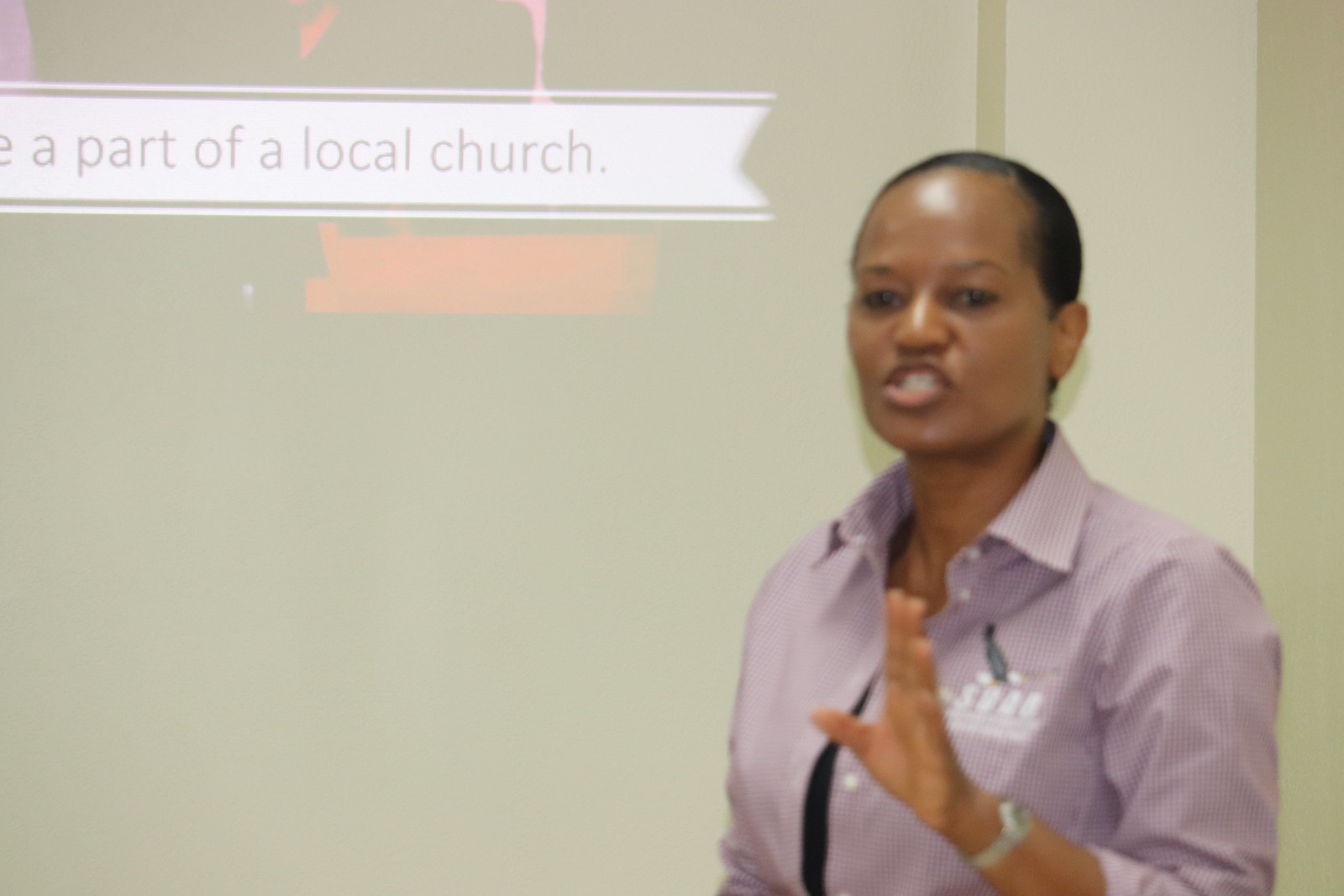A black woman with very short hair passionately addresses an audience in an indoor setting. Positioned in the bottom right corner of the image, she wears a purple collared shirt with a white logo on the left breast, which slightly reveals a black t-shirt underneath, along with a silver wristwatch on her left wrist. Her left hand is raised, palm facing forward, and her mouth is open, showing both the top and bottom rows of her white teeth. The blurry background features a muted grayish-green wall with a horizontal white banner in the upper left corner, partially revealing the text "be a part of a local church." The colors prominent in the photo include purple, white, black, brown, red, pink, and gray. The photograph is a horizontal rectangle, capturing the woman from the waist up as she speaks forcefully in front of the screen.